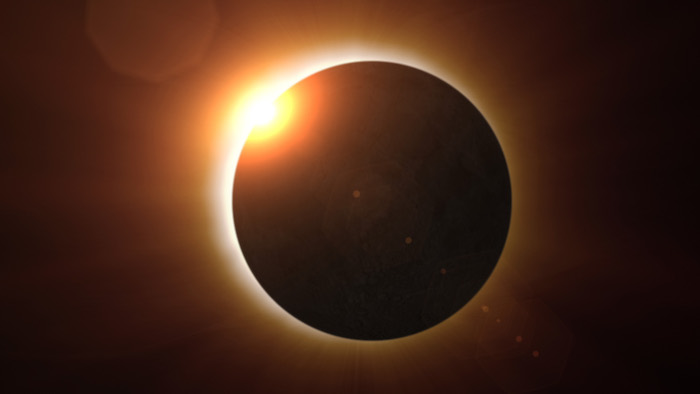In this horizontally aligned rectangular photograph depicting an outdoor scene of a solar eclipse, the moon is positioned to cover almost all of the sun, revealing only a bright yellow sphere of light on the top left corner. The celestial backdrop transitions from dark black to lighter shades, particularly towards the left where the sun’s corona radiates. This corona creates a glowing effect, with a notable orange ring surrounding the yellow-intensity core, ultimately giving way to a white globe of light. The left side of the image exhibits a more brownish tint due to the sunlight, contrasting the near-black darkness on the right. The stark illumination on the left corner forms a distinctive, round reflective spot. Additionally, rays of light stream across the scene, accentuating the intense interplay between the sun and the eclipsing moon. No text is present in the image, which powerfully captures the dramatic moment of the eclipse in a nuanced color palette, ranging from yellow and orange hues to varying depths of brown and black.